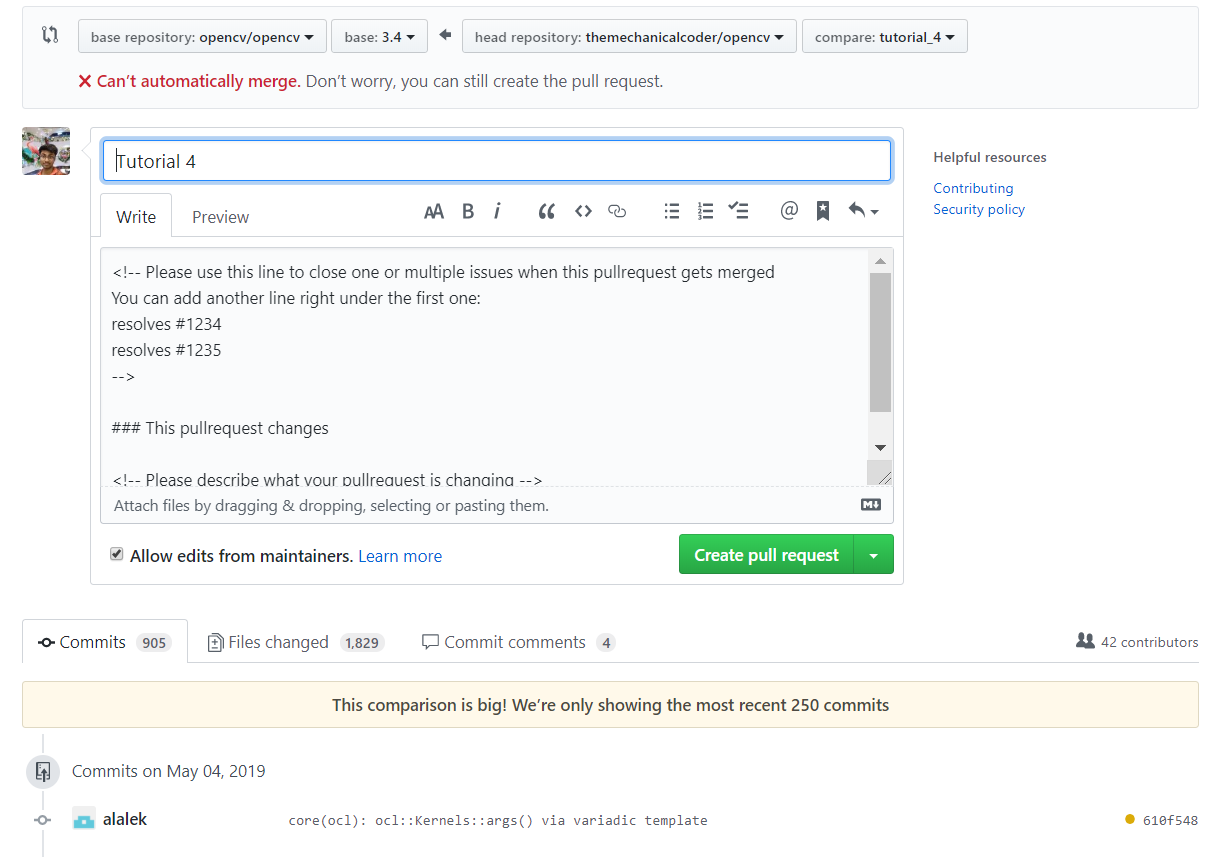Screenshot of a GitHub Pull Request Page:

At the top of the screenshot, there's a header with multiple navigation elements, including drop-down menus. Positioned at the top left corner are two arrows forming a box, followed by four drop-down menus. Directly below these menus, a red text alert reads, "X can't automatically merge," with an additional message to its right stating, "Don't worry, you can still create the pull request."

The main body of the screenshot displays a user profile picture on the left. Adjacent to it on the right is a large white text box titled "tutorial four." Beneath this are tabs labeled "Write" and "Preview," accompanied by icons for formatting text.

Further down, there is another text box for adding additional information. To the far right of this box, a prominent green button labeled "Create pull request" is visible. To the left of this button is a checkbox option with the text "Allow edits from maintainers" and a "Learn more" link next to it.

Below this section, several windows are organized under three tabs: "Commits," "Files changed," and "Commit comments." To the right, there's an icon representing two people, indicating "42 contributors." A yellow box with some information is placed in the center. The area below displays a timeline of commits, starting with "commits on May 4, 2019," followed by the detailed text associated with each commit.